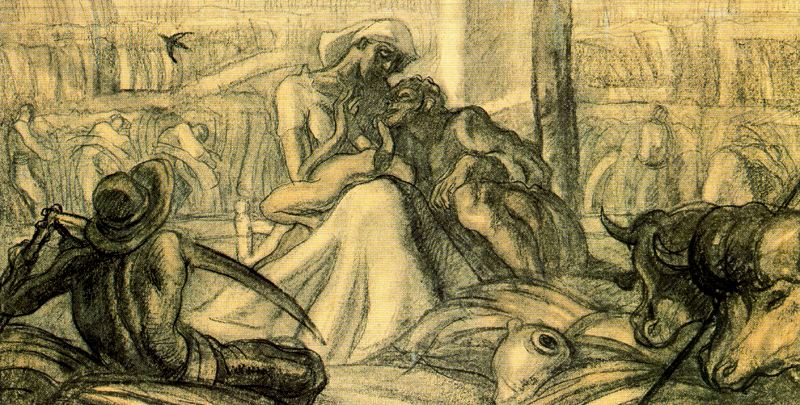In this detailed black and white sketch, a central female figure, resembling a maiden, is depicted breastfeeding a child. She is dressed in a short-sleeved white dress with a white headdress and cloth, her eyes open and right hand raised. Beside her, adding an eerie tone to the scene, is a sinister-looking man who appears disfigured and is also attempting to breastfeed. His unsettling presence is enhanced by his disfigured face and hand draped over his knee. To the right of this central scene, two oxen with downward-facing horns stand prominently in the foreground, enhancing the rustic and impoverished atmosphere. Near the oxen, there's a jug on the ground, while the right-center of the image features a large, eye-like shape with a distinct pupil. On the left side of the foreground, a shirtless man in slacks lounges, holding a scythe or large axe in his left hand, and wearing a cabana hat. The background is fairly nondescript, with sketchy figures that appear to be people either standing upright or leaning, adding a sense of depth and crowd. Additionally, a bird is sketched flying in the upper left corner, and a faint pillar is visible to the right of the central woman, further enriching the intricate scene.